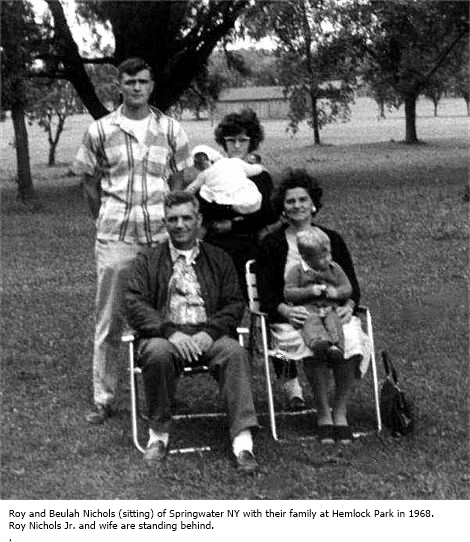A vintage black-and-white photograph from 1968 captures a family gathering at Hemlock Park in Springwater, New York. In the foreground, seated in lawn chairs are Roy and Beulah Nicholas, both appearing to be in their late 40s or early 50s. Roy is wearing a black fall jacket over a plaid button-up shirt, with his hands folded and a bit of gray in his otherwise curly black hair. Beulah, to his right, has dark curly hair, pearl earrings, a black sweater, and a white dress. She is tenderly holding a young boy, likely around three or four years old, dressed in typical young kid attire. 

Standing behind them are their son, Roy Nicholas Jr., and his wife. Roy Jr. is tall, with dark hair parted to the side, a plaid button-up shirt, and light-colored pants, with his arms folded behind his back. His wife, shorter in stature with black curly hair and glasses, holds their baby dressed in a white onesie and a bonnet. Trees and a distant barn frame the scene, reinforcing the rural, farm-like setting. The caption at the bottom of the photograph confirms their identities and the setting: "Roy and Beulah Nicholas of Springwater, New York, with their family at Hemlock Park in 1968. Roy Nicholas Jr. and his wife are standing behind."